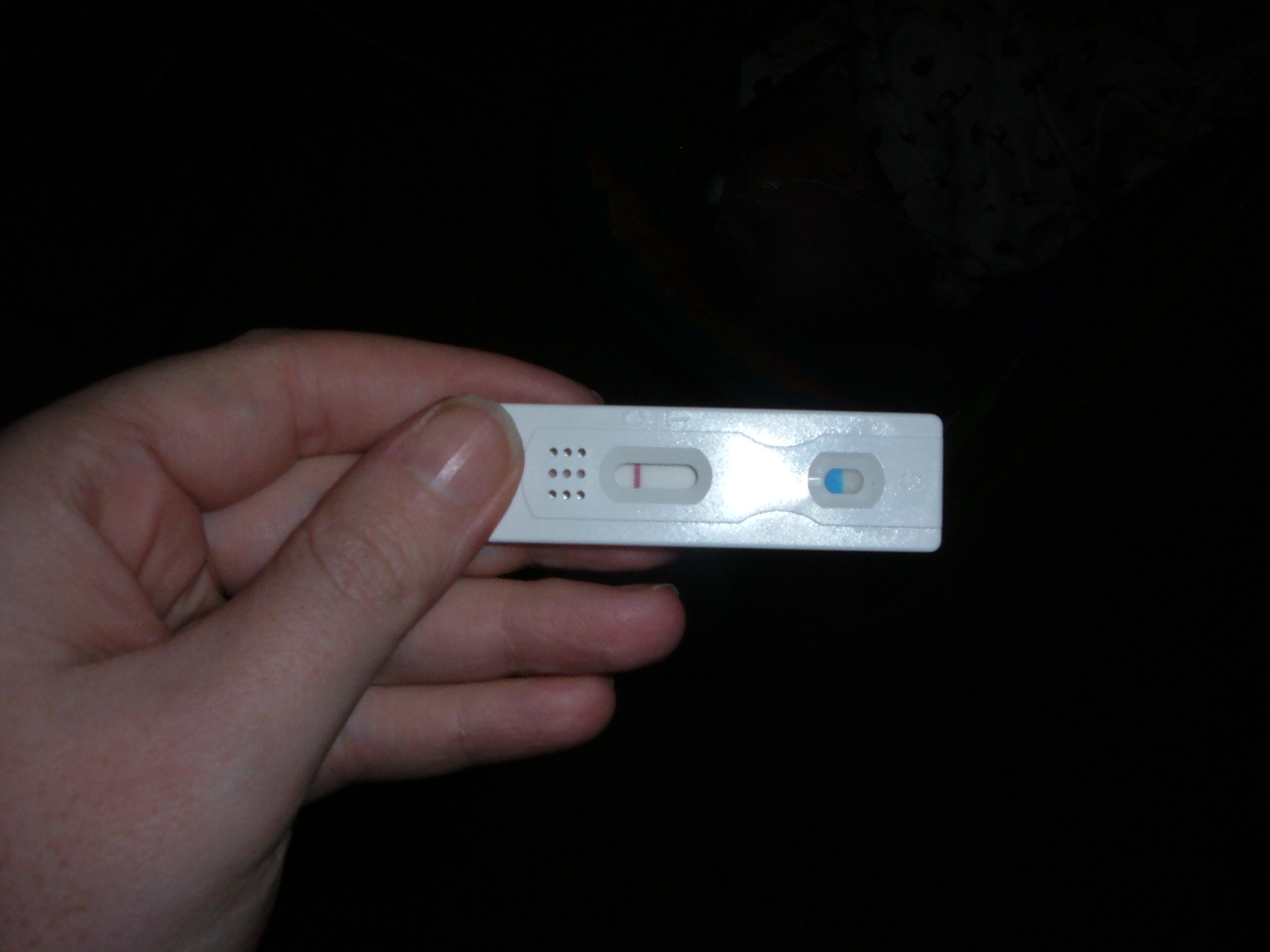Photographed against a completely black background, the focus of the image is a single hand, visible from just below the wrist, suggesting anonymity and universality. The hand, which likely belongs to a younger individual, delicately grasps a rectangular, white pregnancy test. The test features two distinct ovals: one where a line would appear to indicate the result, and another for the urine input. The polished surface of the pregnancy test catches a reflective glare, indicating the use of a light source or camera flash during the photo capture. The thumbnail also reflects this glare, adding emphasis to the meticulous details captured in the image. The hand, potentially feminine, conveys an almost palpable sense of anticipation and emotion, subtly inviting viewers to empathize with the wonder and nervousness surrounding the test's outcome.